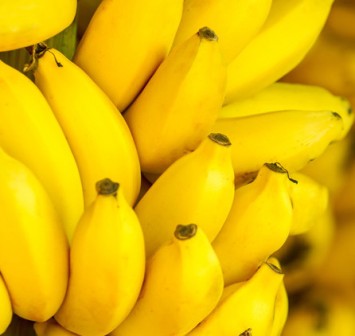This vibrant, close-up photograph captures a cluster of small, wild bananas displayed upside down, their curved yellow forms pointing upwards. The bananas are in sharp focus, showcasing their perfectly yellow skin with only the very tips exhibiting a touch of brown or black discoloration. Featuring around 15 densely packed bananas, the image highlights their pristine freshness and cheerful hue. In the slightly blurred background, the color hints at more bananas. Notably, a bit of green appears in the upper left, possibly from a leaf or trunk of the banana tree, adding a natural context to the scene. One banana displays small, dried strings at its end, emphasizing their authentic, untouched nature.